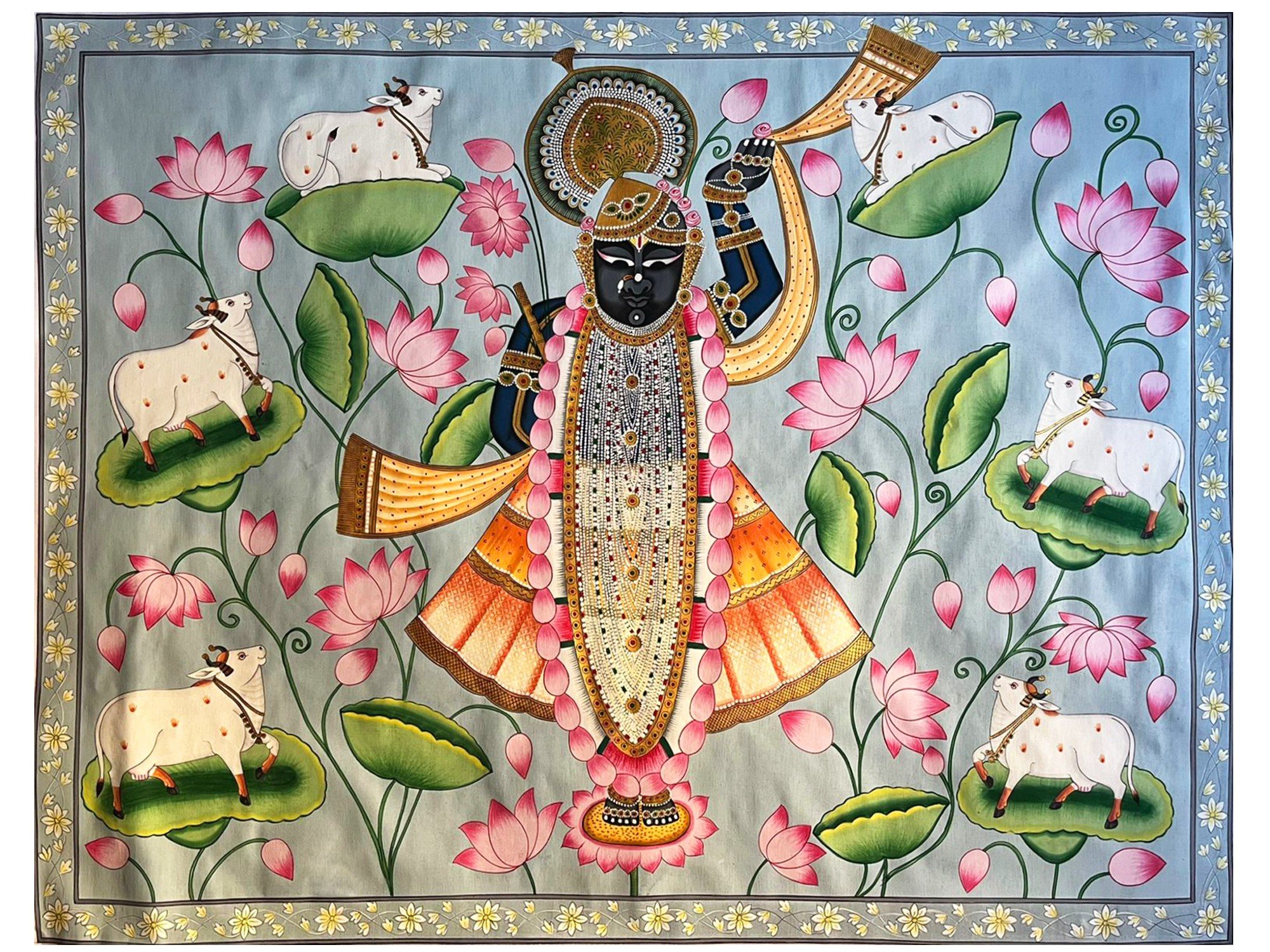In this artwork, rendered on fabric with visible waves along the edges, the primary background color is a gradient of light blue transitioning into a light greenish-yellow hue. Enclosing the central image is a border strip on a bluish-gray background, adorned with intricate floral scrollwork featuring golden beige and yellow flowers with green buds. The border also features white flowers decorating its entire perimeter.

The central figure, set against the bluish cloth backdrop, appears to be an Indian god characterized by black skin. This figure is adorned with elaborate gold bracelets and jewelry, a long, multicolored necklace made of silver and gold that drapes down to the feet, and is depicted with one arm raised, holding a yellow scarf with a brown border, while the other arm extends behind. The figure's head is crowned with an intriguing fan-like headwear, adding to the divine aura.

The god is dressed in an orange skirt that fans out in yellows and oranges, coupled with a detailed, oval-shaped piece with tan-colored beads hanging down to the ankles. Surrounding the figure are large green leaves with pink lotus flowers and thin branches interspersed with white cows situated on the leaves and lily pads. The blend of vibrant colors and cultural elements creates a striking and immersive depiction of traditional Hindu art.